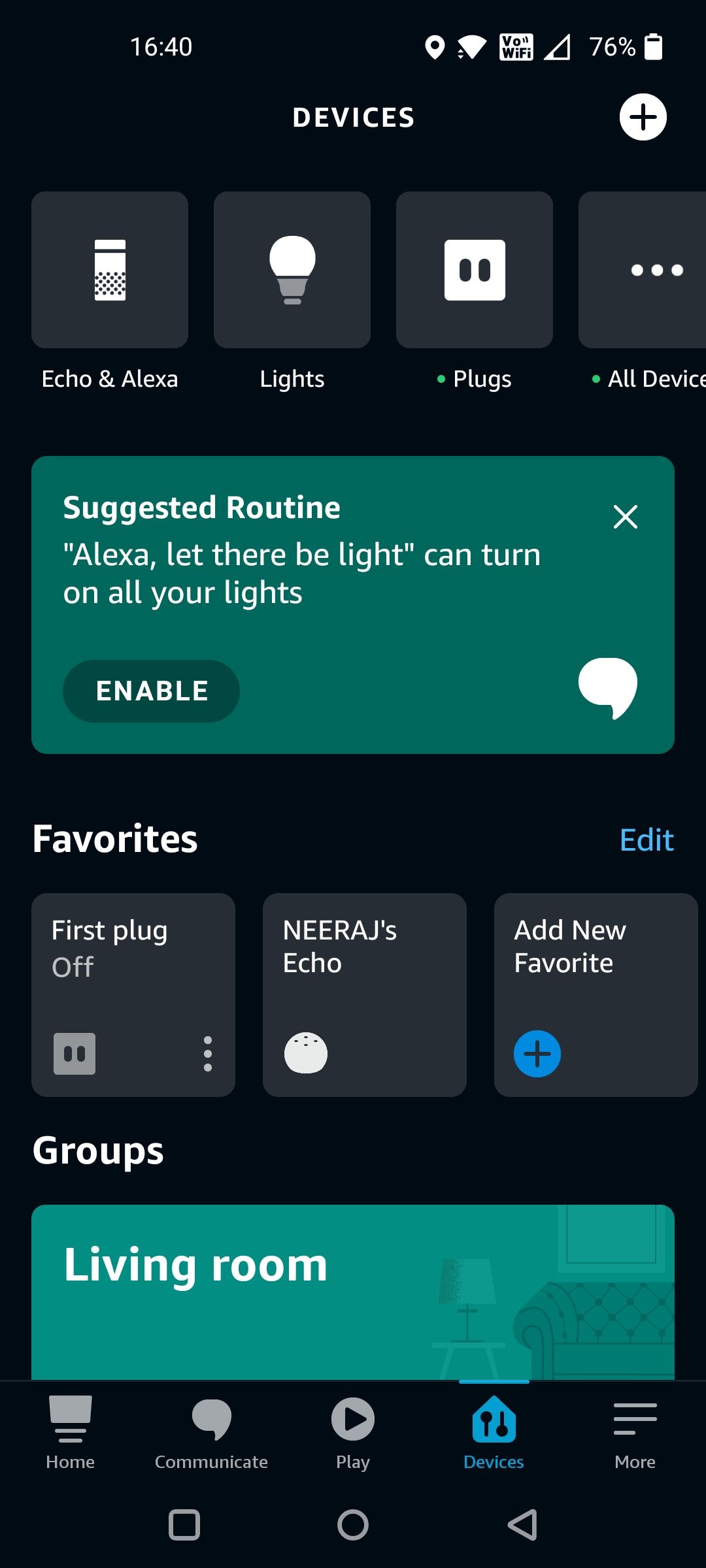The image displayed on the cell phone screen shows a detailed interface of an Alexa-enabled device at 16:40 (4:40 PM) with a 76% battery life and a strong network connection. At the top of the screen, there are gray boxes containing various categories such as "Echo and Alexa," "Lights," "Plugs," and "All Devices," each accompanied by distinct icons. Below these categories, in a green box, is a suggested routine labeled "Let there be light," which can turn on all the lights. There's an "Enable" button next to this feature.

Further down, the "Favorites" section shows "Neeraj's Echo" and an option to "Add New Favorite" in blue with a plus sign. Following this, under "Groups," there is a section labeled "Living Room," highlighted in green with white lettering, alongside an icon of a lamp and a sofa. At the bottom of the screen, there are icons for different functions: "Play," "Communicate," "Home," "Devices," and "More," providing quick access to various features of the device.